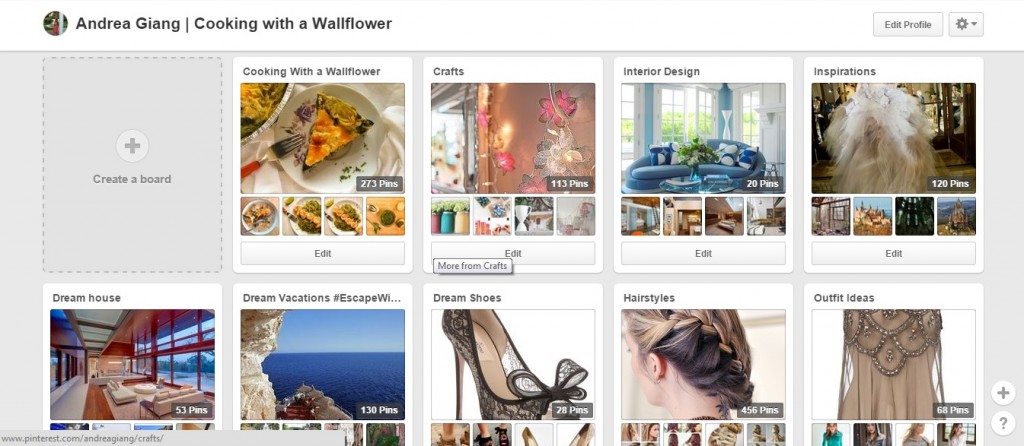**Andrea Jiang’s Pinterest Profile Overview**

**Top Section:**
- **Header:** Features an avatar of Andrea Jiang, followed by a vertical line and "Cooking with a Wallflower" in bold black font.
- **Navigation Bar:** 
  - On the left, a white bar prominently highlights "Edit Profile" with a settings icon featuring a down arrow next to it.
  - Gray background extends behind the dotted gray box containing a plus sign labeled "Create a board".

**Board 1: Cooking with a Wallflower**
- **Primary Image:** A piece of quiche on a plate with a red-handled fork.
- **Board Details:** Contains 273 pins.
- **Additional Images:** 
  - Four smaller images possibly showcasing different dishes like tortellini on plates, although specifics are unclear due to image size.
  - A cutting board with various items including a green round object in the middle, potentially a lime, and some utensils like a spoon or fork.

**Board 2: Crafts**
- **Primary Image:** Light strands adorned with flowers running up a wall.
- **Board Details:** Contains 113 pins.
- **Additional Images:** 
  - Three clay pots with lime-green flowers.
  - Hands crafting with beads (details unclear).
  - A trophy-like cup.
  - Another image of light strands with flowers.

**Board 3: Interior Design**
- **Primary Image:** A blue sofa accompanied by blue and white pillows, arranged in circular patterns. There is a glass-top coffee table holding a blue vase with green and white flowers.
- **Board Details:** Contains 20 pins.
- **Additional Images:** Four smaller images showing various interior design concepts, though specific details are not clear due to image size.

**Board 4: Inspirations**
- **Primary Image:** Flowing white material resembling wedding veils or ghostly fabric with a brown undertone, set in a room with glass display cases.
- **Board Details:** Contains a few inspirations.
- **Additional Images:** 
  - A castle with a scenic mountain view.
  - Another castle on a hill.
  - A side building.

**Board 5: Outfit Ideas**
- **Primary Image:** A brown dress with glittery stones on the bodice.
- **Board Details:** Contains 68 pins.
- **Additional Images:** Four smaller images of various women's fashion items, including teal and white outfits.

**Board 6: Hairstyles**
- **Primary Image:** A French braid descending diagonally down the back of a person's head, who has a neck tattoo.
- **Board Details:** Contains 45 pins.
- **Additional Images:** Various hairstyle ideas.

**Board 7: Dream Shoes**
- **Primary Image:** A lacy black stiletto with a lacy bow on the front.
- **Board Details:** Contains several images of shoes.
- **Additional Images:** Four more pairs of stylish shoes.

**Board 8: Dream Vacations**
- **Primary Image:** A picturesque waterfront setting featuring a rock wall on the left, with a pier structure in the shape of a boat harboring four umbrella-topped tables alongside a beautiful blue ocean backdrop.
- **Board Details:** Contains 130 pins.
- **Additional Images:** Four smaller vacation spots.

**Board 9: Dream House**
- **Primary Image:** An elongated view of a room with windows on both sides. The living room has a couch and a perpendicular lounge chair with a round white coffee table. Beyond this area is what appears to be a kitchen with a bar. The room features wooden floors and gray carpeting running adjacent to a walkway, with wooden columns extending to the roof.
- **Board Details:** Various dream house inspirations.

**Footer:**
- A gray bar at the bottom includes the web address: www.pinterest.com/AndreaJiang/crafting, depending on where the cursor is resting.